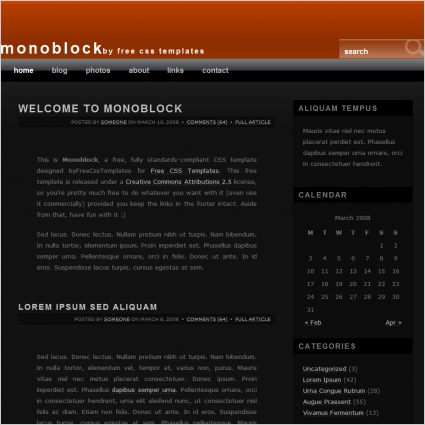The image is a blurry screenshot of a website featuring a template called "Monoblock" by Free CSS Templates. The layout includes a rust-colored header with the title "Monoblock" prominently displayed alongside a search box. Below the header, there is a navigation menu with the options: "Home," "Blog," "Photos," "About," "Links," and "Contact." The background is black with white text. The main headline states "Welcome to Monoblock" followed by placeholder text "Lorem ipsum sed aliquam." On the right side of the image, there is a section displaying a calendar for March 2008 and a list of categories including "Uncategorized." The template is described as fully standards-compliant and available under a Creative Commons Attribution 2.5 license, allowing for free use as long as the footer links are kept intact.